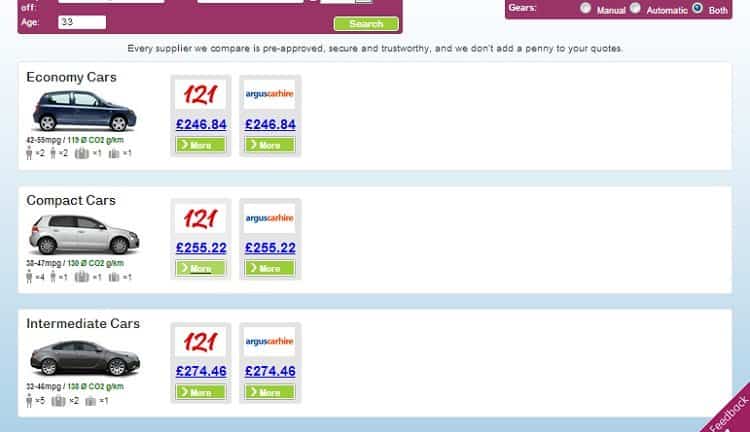The screenshot shows a car rental website with a dark purple header featuring a small age input box displaying "33." Alongside is a green search bar positioned near the center. The far-right section of the header includes three radio buttons for selecting gearbox options: Manual, Automatic, and Both, with "Both" currently selected. The website's title reads, "Every supplier we compare is pre-approved, secure, and trustworthy. We don't add a penny to your quotes."

Below the header, the page is divided into three sections showcasing car types with accompanying details:

1. **Economy Cars**:
   - Capacity: 2 people or 4 (2 people per car), 1 luggage
   - Fuel Efficiency: 55 miles per gallon
   - Price: Starts at 246.84 euros on both One-to-One and Arcus Car Hire websites.

2. **Compact Cars**:
   - Price: Fixed at 255 euros on both One-to-One and Arcus Car Hire websites.

3. **Intermediate Cars**:
   - Price: Fixed at 274.46 euros on both One-to-One and Arcus Car Hire websites.